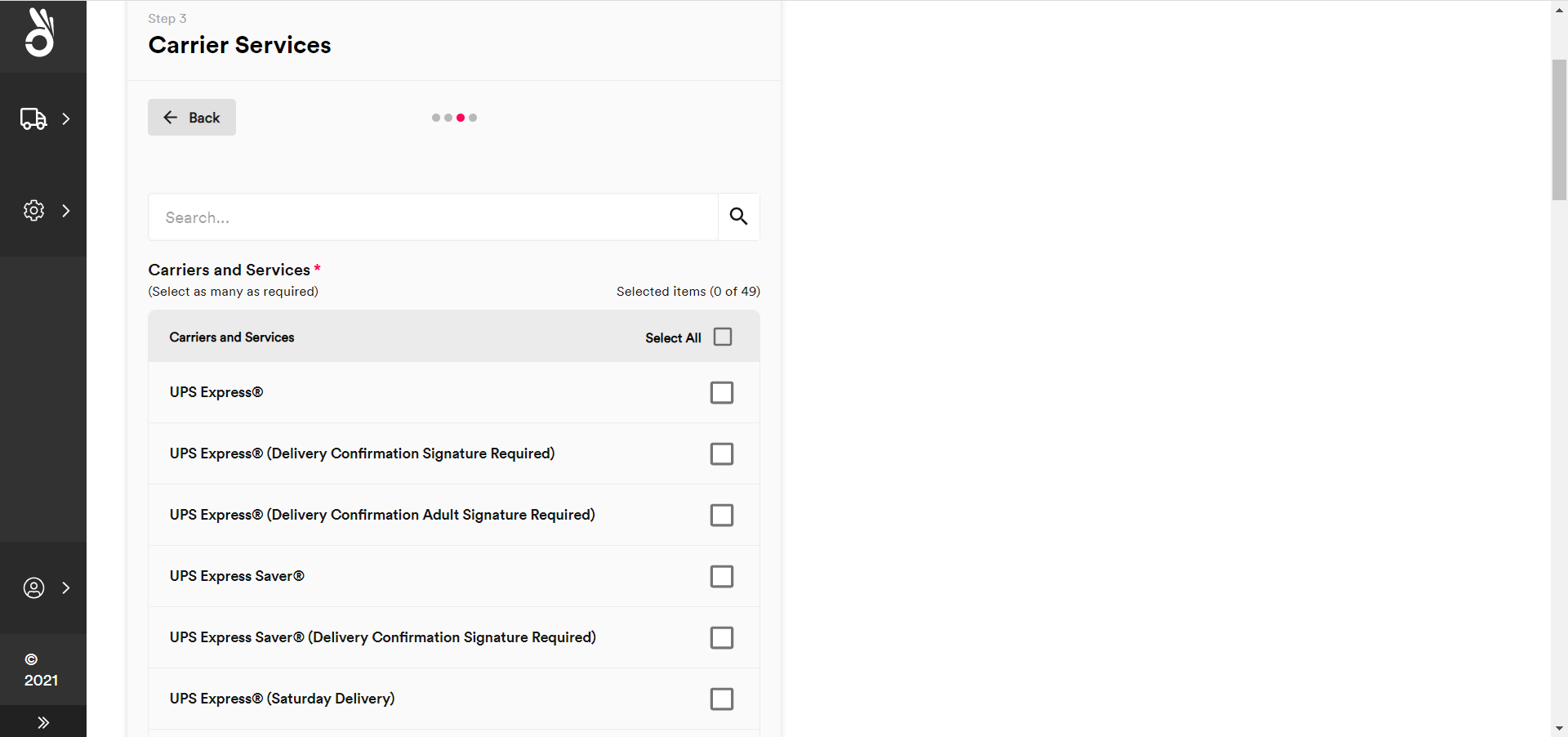The monochromatic web page features a black vertical panel on the left side, displaying a white symbol resembling the "OK" hand gesture—where the index finger and thumb form a circle and the remaining three fingers are extended. The panel includes several interactive icons: an icon of a delivery truck to open a tab, a settings icon with another tab, and a profile icon at the bottom, also with a tab. Additionally, the bottom of this panel displays the text “Copyright 2021” along with two arrows.

At the top of the main content area, "Step 3" is written in small gray text, while "Carrier Services" appears prominently in larger black font. A gray back button featuring an arrow is present, and three bubbles are visible, one marked with a red icon. Near the top, there is a search button symbolized by a magnifying glass.

Below these elements, the section labeled "Carriers and Services" has a red asterisk next to it, indicating a required field. The instruction "Select as many as required" is provided, along with a gray button labeled "Carriers and Services. Select all." Following this, "UPS Express" is listed, accompanied by an interactive button.